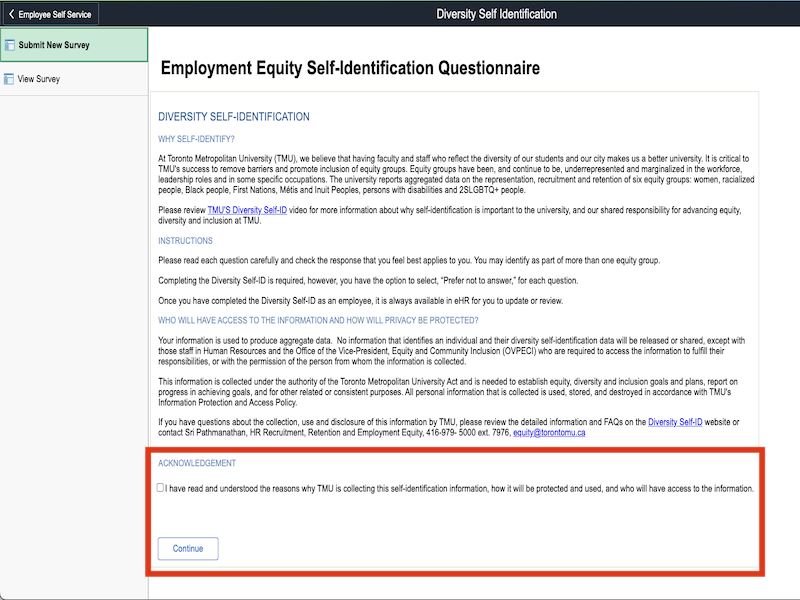This is a close-up screenshot of the Diversity Self-Identification webpage from Toronto's Metropolitan University. The webpage features a comprehensive Employment Equity Self-Identification Questionnaire divided into several sections, each adorned with blue headings and black descriptive text. 

The first heading, "Why Self-Identify," explains the university's commitment to reflecting the diversity of its students and community, emphasizing the importance of inclusive practices to the institution's success. It highlights the university's aim to dismantle barriers and promote equity among six specific groups: women, racialized people, Black individuals, First Nations, Métis and Inuit people, persons with disabilities, and 2SLGBTQ+ individuals. It mentions the university's practice of reporting aggregated data on these groups' representation, recruitment, and retention.

Beneath this heading, there is a prompt to watch TMU's diversity self-identification video for more information on the significance of this initiative and the shared responsibility for advancing equity, diversity, and inclusion at TMU. Further instructions and privacy protection details are provided below.

There are other sections on the webpage with headings such as "Instructions," "Who Will Have Access to the Information and How Privacy Will Be Protected," and "Acknowledgement." The "Acknowledgement" section allows users to confirm their understanding of how their information will be used and protected before proceeding by ticking a checkbox and clicking "Continue."

On the left side of the webpage, two navigation options, "Submit New Survey" and "View Survey," are present. The "Submit New Survey" option is currently selected, indicated by a green background.